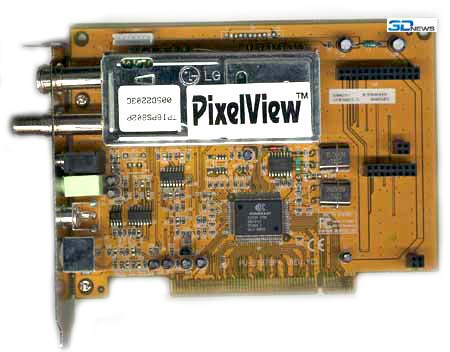The image features a brown computer chip resembling the color of wood. Prominently displayed on this chip is a silver contraption, or box, topped with a white label. The label bears the logo "PIXLVIEW" accompanied by a trademark symbol next to the "W" in "VIEW". To the left of the PIXLVIEW label, there is another white label, which is positioned upside down, making its digits challenging to read. The upper right corner of the brown computer chip is marked with the text "3DNEWS". The intricate arrangement and the mix of distinct labels suggest a detailed and specialized piece of technology.